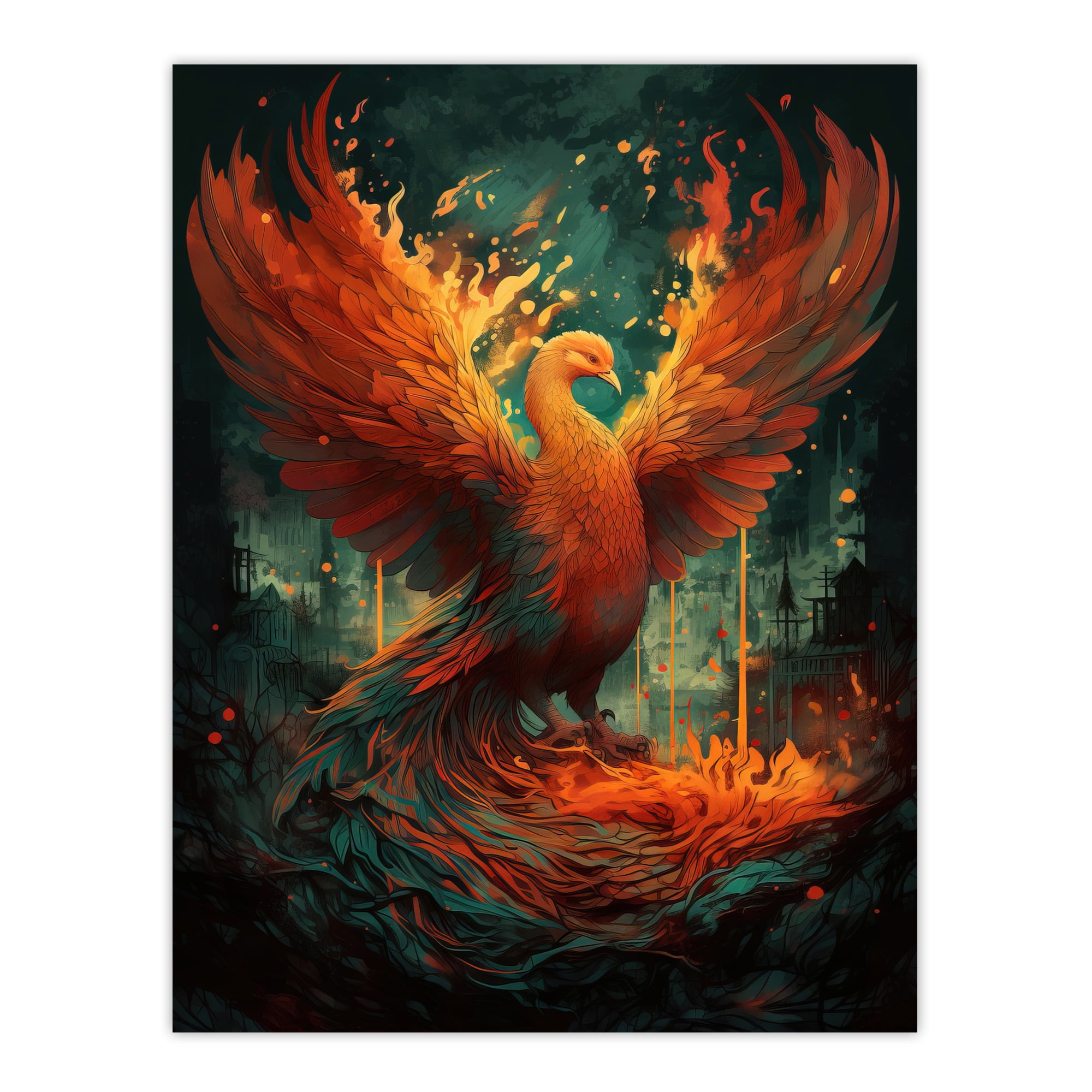An intricate, animated phoenix dominates the foreground of this captivating illustration. The phoenix is vividly depicted with a vibrant mix of bright orange and yellow feathers that appear to be ablaze, creating a mesmerizing display of fiery wings spread wide across the image. Its majestic head arches down to a gracefully curving body, transitioning into blue feathers that cascade towards its long tail, which wraps around the bottom of the artwork. The tail's blue hue melds back into a fiery orange at the tips, mirroring the wings. The bird's claws are distinctly visible, adding to its imposing presence. Behind the phoenix, the background features a dark, blackish-blue gradient with faint, old buildings and a tree to its left, emphasizing the bird as the striking focal point against the shadowy cityscape. The artwork's meticulous detail and dynamic colors bring the mythical creature to life in a dramatic and enchanting manner.